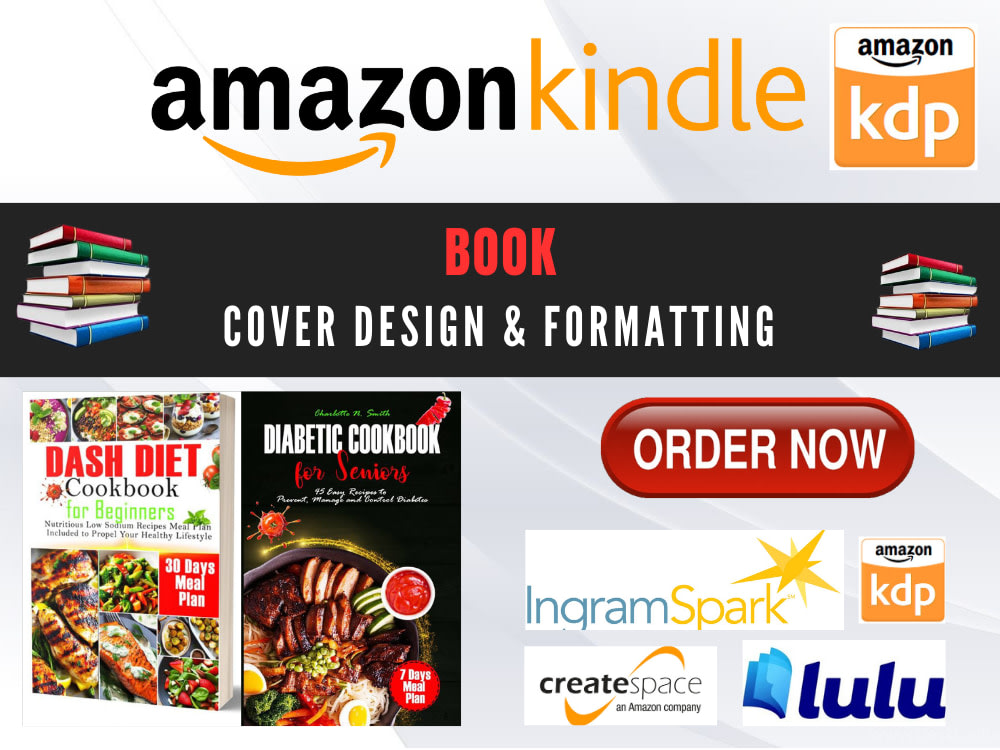The image is an advertisement for Amazon Kindle. At the top, against a white and gray background, the black Amazon logo is accompanied by the orange smile underneath, along with the word "Kindle" in orange. To the right, there's a small square with the Amazon KDP logo—Amazon in black on a white background and "KDP" in larger white letters on an orange background. Beneath this, a black strip features the word "book" in red and "cover design and formatting" in white, with stacks of book illustrations on either side, showcasing various colors like red, green, orange, and blue.

Below this band, on the left side, are two cookbook covers: one titled "DASH Diet Cookbook for Beginners" with a '30 days meal plan' label and an array of food images, and the other titled "Diabetic Cookbook for Seniors" featuring a dish in a skillet on a black background. To the right of these covers, there is a prominent red button with white text that reads "order now." Underneath the button, a series of logos from IngramSpark, Amazon KDP, CreateSpace, and Lulu are displayed, indicating the platforms available for book design and publishing.